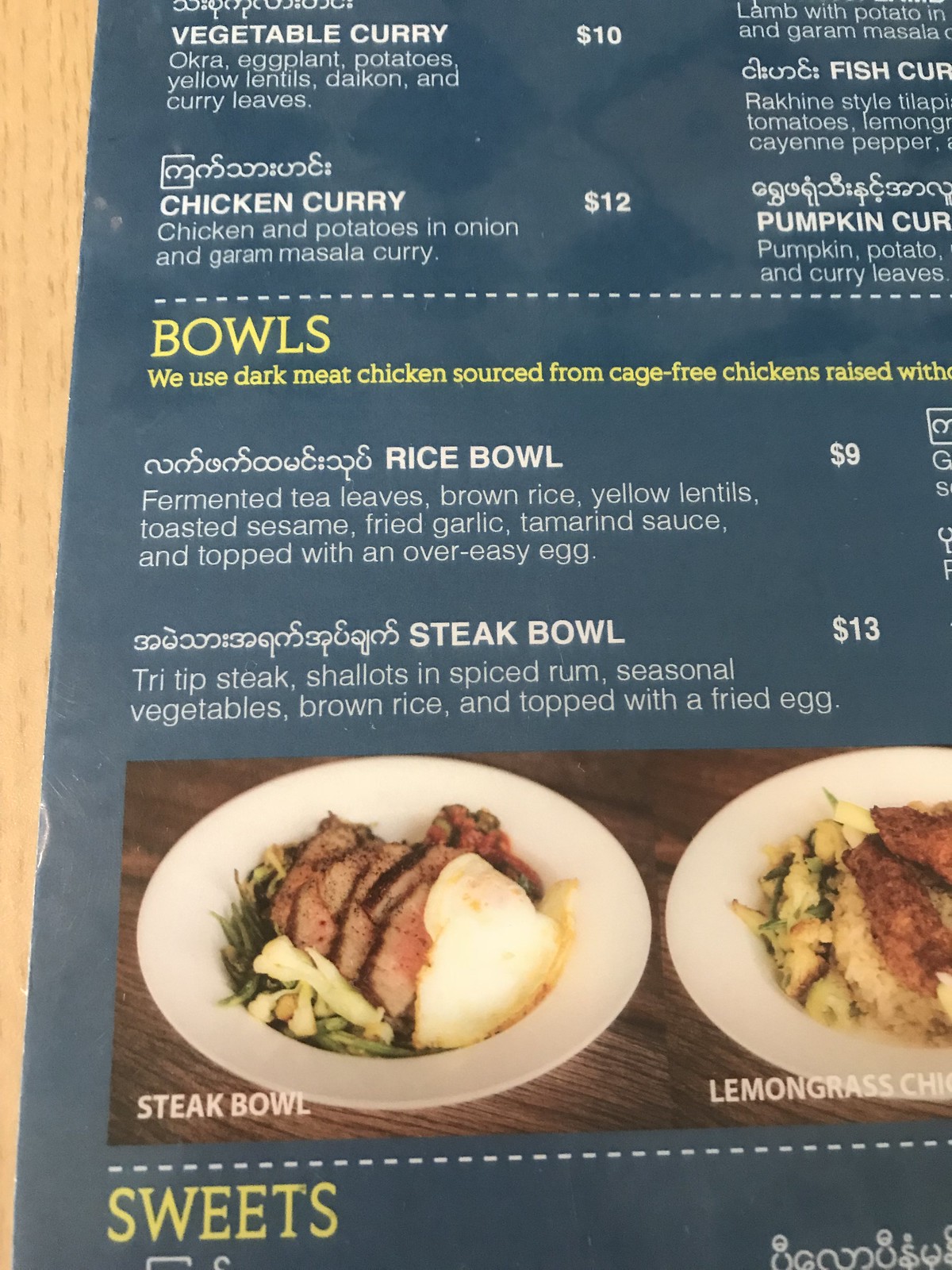The image displays a page from a menu placed on a light pinewood surface. The menu page features pictures of two meals: the dish on the left is labeled "Steak Bowl," while the dish on the right is labeled "Lemongrass Chicken."

At the top of the menu, the following items are listed:
- **Vegetable Curry** - $10: Consists of okra, eggplant, potatoes, yellow lentils, daikon, and curry leaves.
- **Chicken Curry** - $12: Contains chicken and potatoes in an onion and garam masala curry.

In a section marked in yellow labeled "Bowls," the menu describes:
- **Rice Bowl** - $9: Includes fermented tea leaves, brown rice, yellow lentils, toasted sesame, fried garlic, tamarind sauce, and is topped with an over-easy egg.

Additionally, the menu notes that the chicken used is sourced from cage-free chickens raised without the use of certain unethical farming practices.